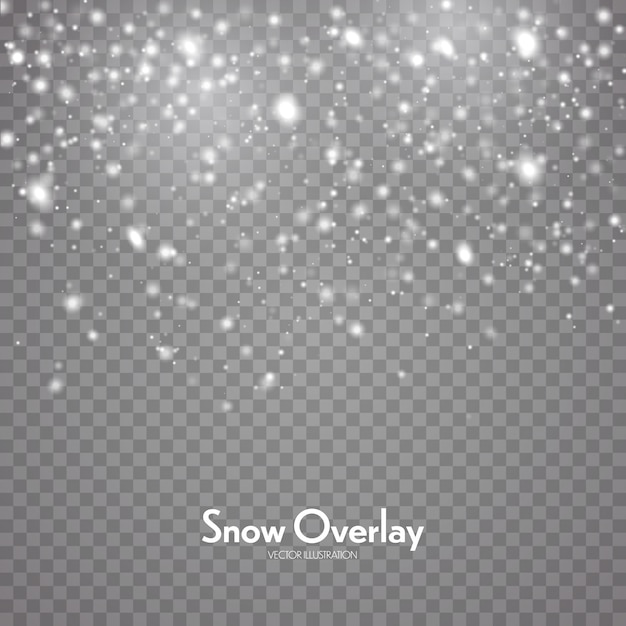The image features a subtle checkerboard background composed of tiny, alternating squares in lighter and darker shades of gray. The upper half of the scene is interspersed with various white starburst shapes and specks that increase in density toward the top, suggesting a snowfall effect. These white specks appear to glow slightly, surrounded by faint halos, contributing to an illuminated appearance. At the bottom center, the text "snow overlay" is prominently displayed in a white font, with "VECTOR ILLUSTRATION" in smaller, all-capital letters beneath it, both blending seamlessly with the overall gray and white color scheme.